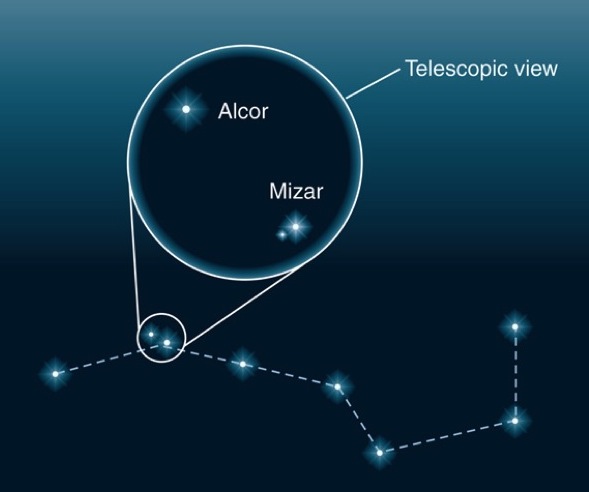This image is a color illustration depicting a stylized constellation against a gradient background that transitions from dark blue at the bottom to a lighter teal at the top. The main feature is a diagram of the Big Dipper constellation, portrayed with bright stars connected by dotted gray lines to outline its distinctive ladle-like shape. The handle of the Dipper starts on the left, and the scoop extends to the right. A focal point of the illustration is a circular inset near the second star from the left in the Dipper's handle. This inset, highlighted by a blue circle, provides a telescopic view showing two stars, Alcor and Mizar, in greater detail, with Alcor positioned at the top left and Mizar at the bottom right of the circle. A white line connects this inset to the main diagram, and a label in white text reads "Telescopic View."